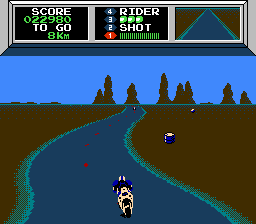A still from an 8-bit motorcycle racing game showcases a digital desert landscape. The top corner of the screen features a progress bar with a large silver display box divided into three sections. On the left side of the display, "Score" is written in white, showing a score of 022980 in green. Located below is the text "To Go," also in white, indicating 8 kilometers in green.

In the center of the display are vertically arranged numbers: 4, 3, 2, and 1. Numbers 4, 3, and 2 are presented in blue with white text, while number 1 is red with white text, all set against a black background. Number 4 is labeled "Rider"; number 3 has three green dots; number 2 is labeled "Shot"; and number 1 contains a health or progress bar depicted with vertical green lines.

On the right-hand side of the display, a digital image of a twisted, dark blue road stretches across the desert landscape. The road has two straight lanes with a blue center and aqua lines along the sides, bordered by brown terrain. Red stripes adorn the middle of the road. In the far background, stone pillars dot the horizon.

One racer is visible on the road, clad in blue armor with a white helmet featuring a blue stripe. The racer rides a white motorcycle with a black back tire. On the brown landscape, a blue oil barrel stands upright on the right side of the screen, while another barrel appears to be lying on its side in the distance.